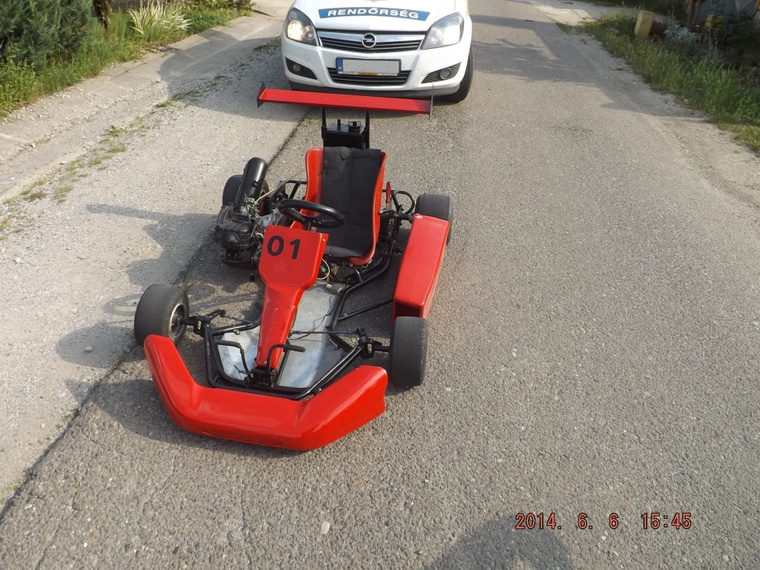In this detailed scene captured on June 6, 2014, at 15:45, a small red go-kart with the number 01 prominently displayed on its frame sits on a grey asphalt road, surrounded by patches of grass and trees on either side. The go-kart features a red exterior, complemented by a black seat and steering wheel. Behind the go-kart, a white car with the word "RENDŐRSÉG" on the hood, suggesting it is a police car, has its headlights turned on. The car's long license plate is indistinguishable in the image. The road appears slightly weathered, with some grass sprouting from the cracks. The clear, sunlit day further emphasizes the natural surroundings, depicting a typical summer afternoon. Notably, the absence of people in the frame heightens the focus on the stationary go-kart and the white car in what seems like an unusual roadside encounter. The image, likely a frame from a camcorder considering the timestamp in the bottom right corner, captures this intriguing moment with striking clarity.